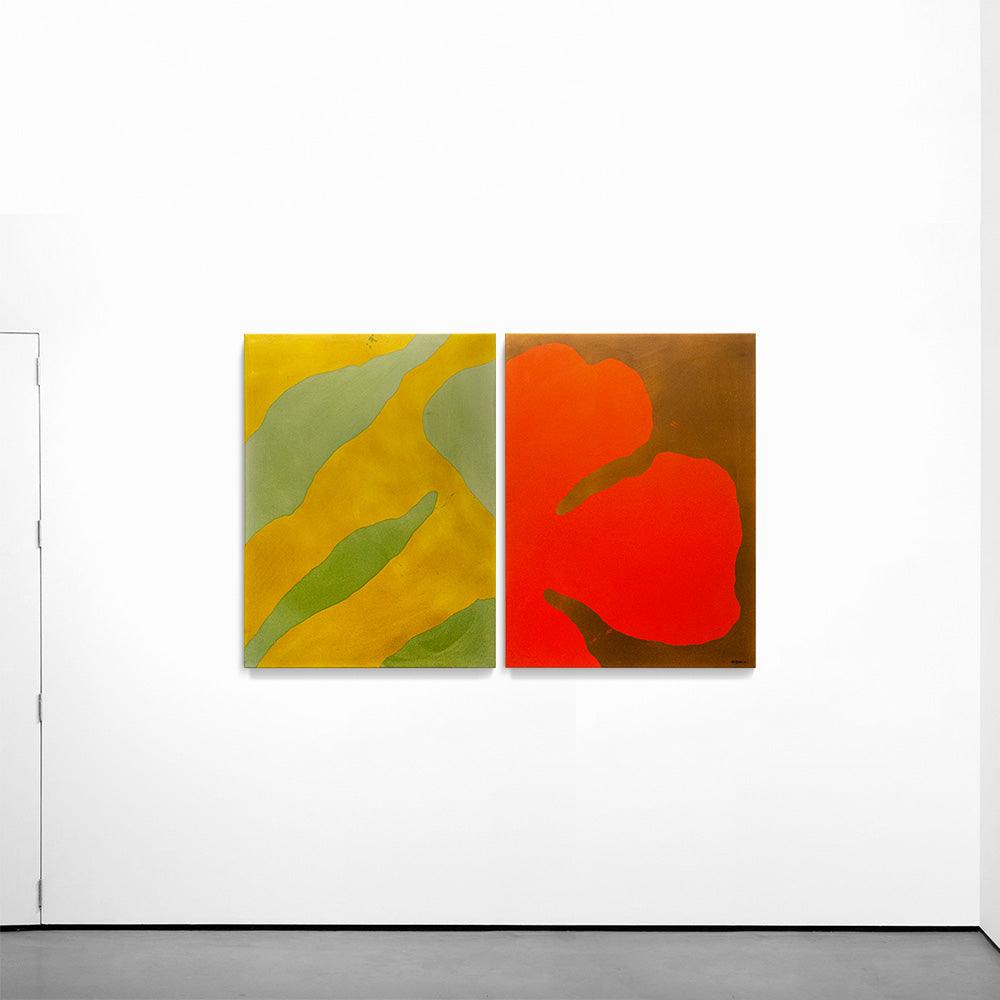The image portrays a section of an art gallery with stark white walls and a gray concrete floor. On the left-hand side, you can discern the outlines and hinges of a partially visible door. Dominating the central focus of the image are two vertically rectangular canvases, each approximately four feet tall, hanging side by side in a symmetrical arrangement. The painting on the left features elongated shapes in green and gold hues against a yellow background, possibly representing abstract leaves. In contrast, the painting on the right displays a red shape akin to a flower or its petals set against a brown backdrop. Together, the vibrant colors of the artwork provide a striking contrast to the minimalist white walls and gray floor of the gallery space.